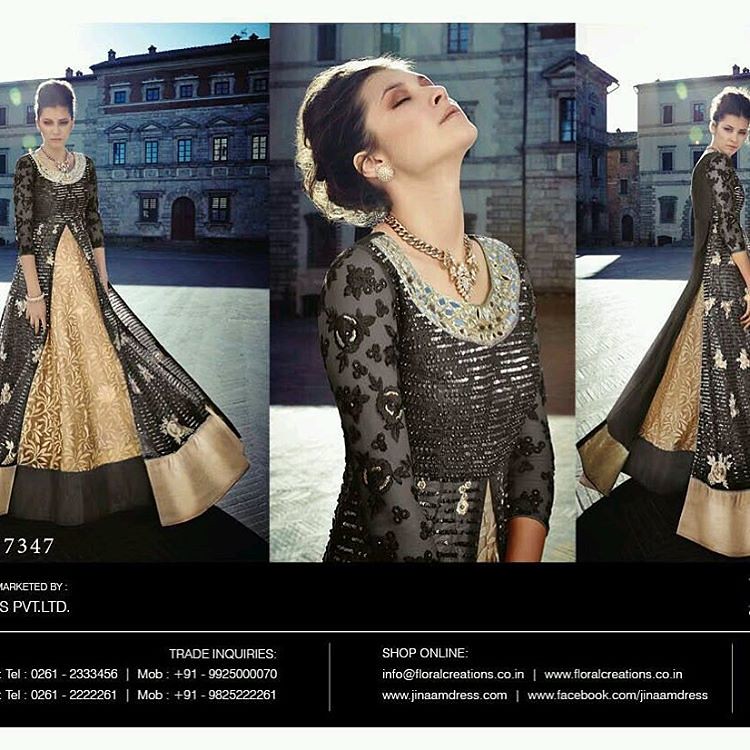The image is a detailed commercial advertisement, formatted as a three-paneled color photograph often seen in high-end clothing catalogs. It features a model with dark brown hair, styled in a bouffant look with her hair tied up around the back of her neck. She is modeling a luxurious, Renaissance-inspired gown that is primarily brown and gold, with intricate detailing. The full-length dress has a scoop neck adorned with a thick, embroidered detail, three-quarter sleeves, a corseted bodice, and panels of gold and brown fabric. The skirt of the gown is partially covered in embroidered netting with glittery accents, and the opaque sleeves showcase a stylized floral pattern. In the left panel, the model stands in a Mediterranean-style palazzo, directly facing the camera, allowing a clear view of the front of the dress. The middle panel offers a closer profile view of her face, eyes closed as she seems to bask in the sunlight, highlighting her striking golden earrings and a detailed double-knot gold necklace with a central pendant. The right panel captures her in a side profile, displaying the back and side detailing of the dress, including the underskirt and overskirt. 

Along the bottom inch of the image is a black rectangle with white text. The left side of this rectangle details "MARKETED BY SPVT LTD" and "TRADE INQUIRIES" with phone numbers listed underneath. The right side displays "SHOP ONLINE" with corresponding email addresses and website links, some indicating availability on Facebook or the Creations Company's online site. This professional layout ensures that potential customers can easily access purchase information.